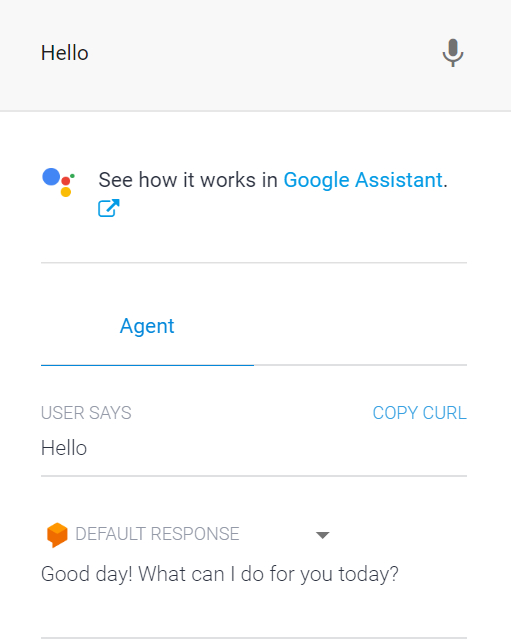A digital screenshot is displayed, featuring various interactive elements related to Google Assistant. At the very top of the image, the word "Hello" is prominently shown. To the right of this greeting, there is a grey microphone icon symbolizing voice input capabilities. Below this, a prompt reads, "See how it works in Google Assistant," inviting users to explore its functionalities.

Central to the screenshot is a set of colorful circular icons: a large blue circle, a smaller red circle, an even smaller yellow circle, and a tiny green dot, which likely represent the Google Assistant's visual identity.

Beneath these icons, the word "Agent" appears in blue, which is underlined by a line that starts off blue on the left and transitions to grey as it extends to the right. This line separates the agent's section from the user's input.

In the user input section, it says "Hello," indicating a greeting or an initial interaction. The text "Copy curl" follows, rendered in uppercase grey, possibly referencing a command or function code. An orange box frames this section, highlighting it.

Below the orange box, the assistant's response begins with a friendly "Good day!" followed by an inquiry, "What can I do for you today?" This warm and inviting response is followed by a long straight grey line at the very bottom of the screenshot, which likely serves as a divider between messages or sections.

Overall, the screenshot captures a structured and user-friendly interface of the Google Assistant, showcasing its various interactive elements and a welcoming tone.